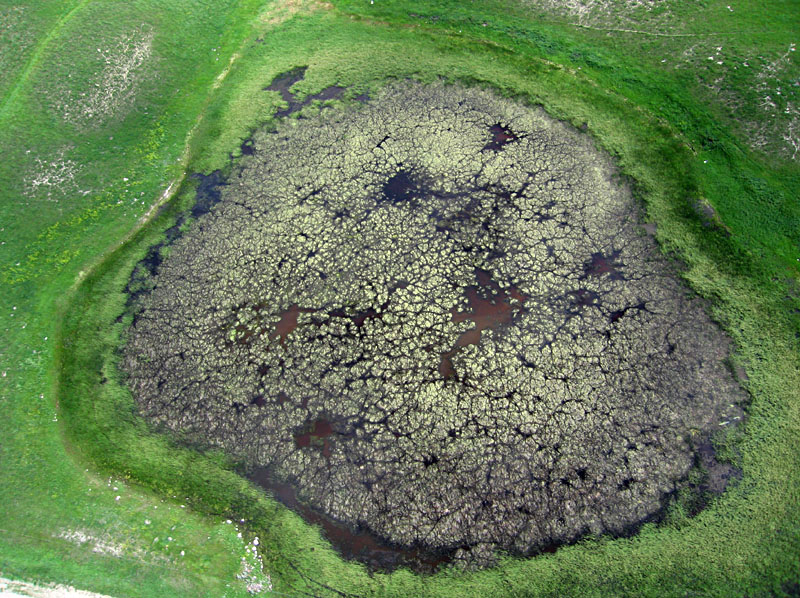This aerial photograph captures a small, irregular-shaped pond, heavily encrusted with algae and plant growth. At the center of the pond lies dark, murky water, intermittently visible through patches where the algae are sparse. The central water exhibits an array of colors, from dark black to brownish-red, often described as uninviting and reminiscent of pollution.

Surrounding the central water, the algae form concentric rings with varying shades of green—from vibrant light green to darker, grayish-green—blending into a white, filmy texture in some areas. The algae create a fuzzy, uniform appearance, with certain thicker regions where the water underneath is completely obscured.

The pond is bordered by patches of green grass interspersed with areas of bare dirt and rocks, especially visible in the upper left, upper right, and bottom left corners of the image. This grassy perimeter transitions from lighter green close to the water to darker green as it moves outward. The overall scene is natural, devoid of any signs of human habitation or structures, giving a sense of secluded wilderness.